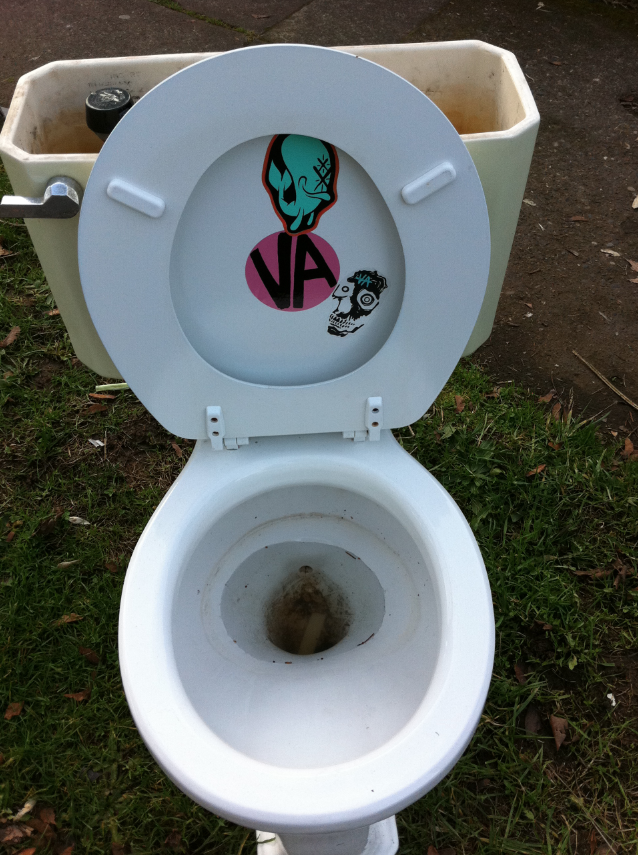The photo captures a strikingly out-of-place scene of a porcelain toilet set in a natural outdoor environment during the daytime. The camera faces downward, revealing the ground beneath the toilet, which transitions from a grassy area adorned with dead leaves at the bottom to a muddy path stretching from the top right to the top left corner. The toilet's white seat is upright, prominently displaying three stickers: a green cartoon whale, a pink circle with the black initials "VA," and a jungle-themed face with large eyes and teeth. The water tank, uncovered and yellowed with age, houses a black water pump and a silver lever. Both the bowl and the tank contain murky water, hinting at disuse and neglect. The tank interior also exhibits signs of rust, adding to the overall dilapidated appearance. A concrete path lies behind this unusual setup, further highlighting the toilet's odd placement in an otherwise natural setting.